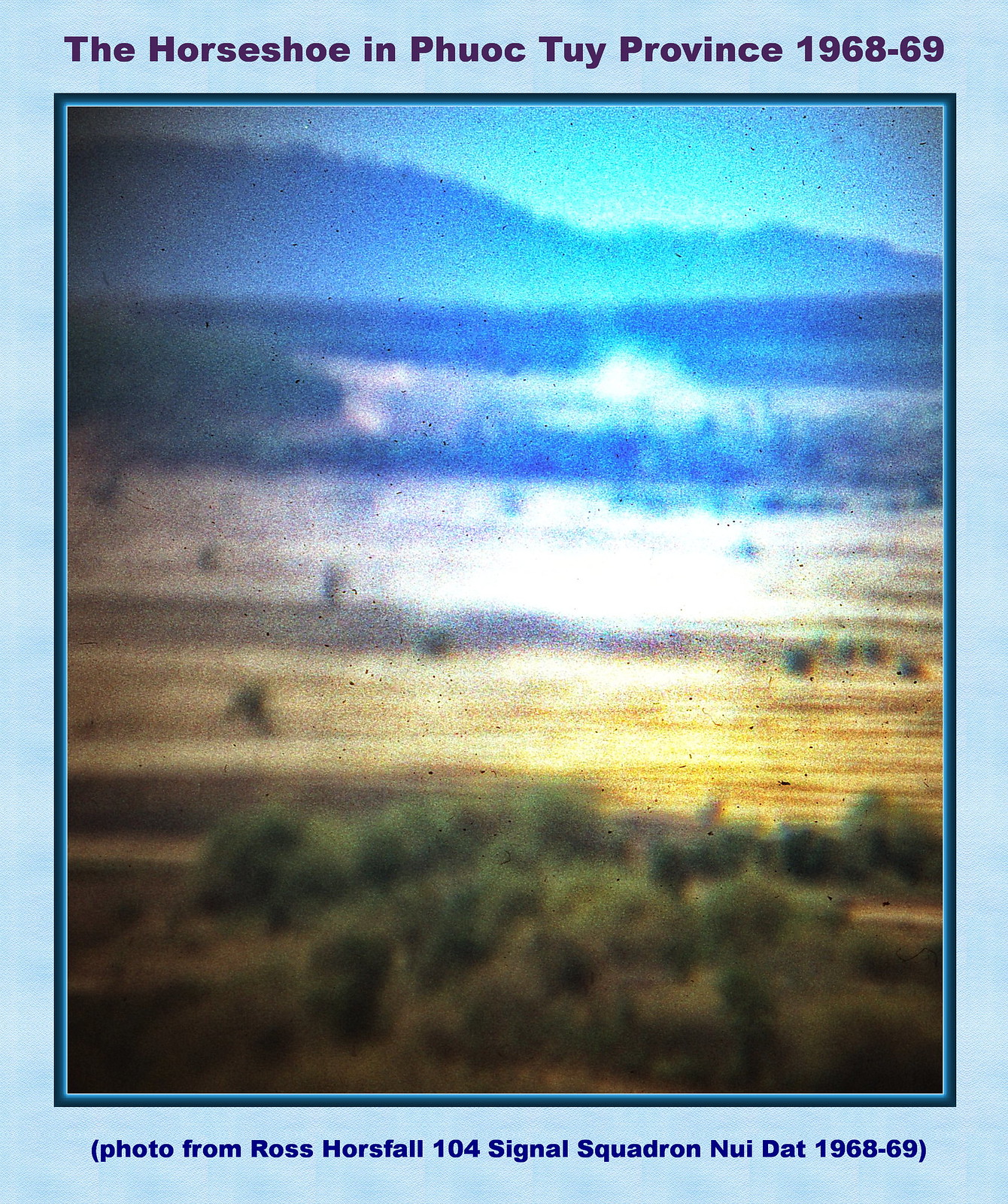This image is a photograph, though the resolution is exceedingly poor, rendering it almost indistinguishable. Only general colors and shapes can be perceived through the graininess and black specks scattered across the photo, suggesting possible damage during capture. The photo appears to depict a distant landscape scene. At the top, there is likely a sky with shades of blue. The middle section features large areas of sandy or open ground, with sporadic patches of greenery implying the presence of trees or low bushes. The bottom part shows prominent hills adorned with trees and additional greenery. The overall landscape suggests a natural setting, possibly with some atmospheric haze or smoke in the distance hinting at an explosion or disturbance. This image is encased in a light blue border, with text at the top stating "The Horseshoe in Phuoc Toi Province, 1968-69" in purple, and a caption at the bottom within the border reading "A photo from Ross Horse Fall 104 Signal Squadron, Nui Dat, 1968-69."